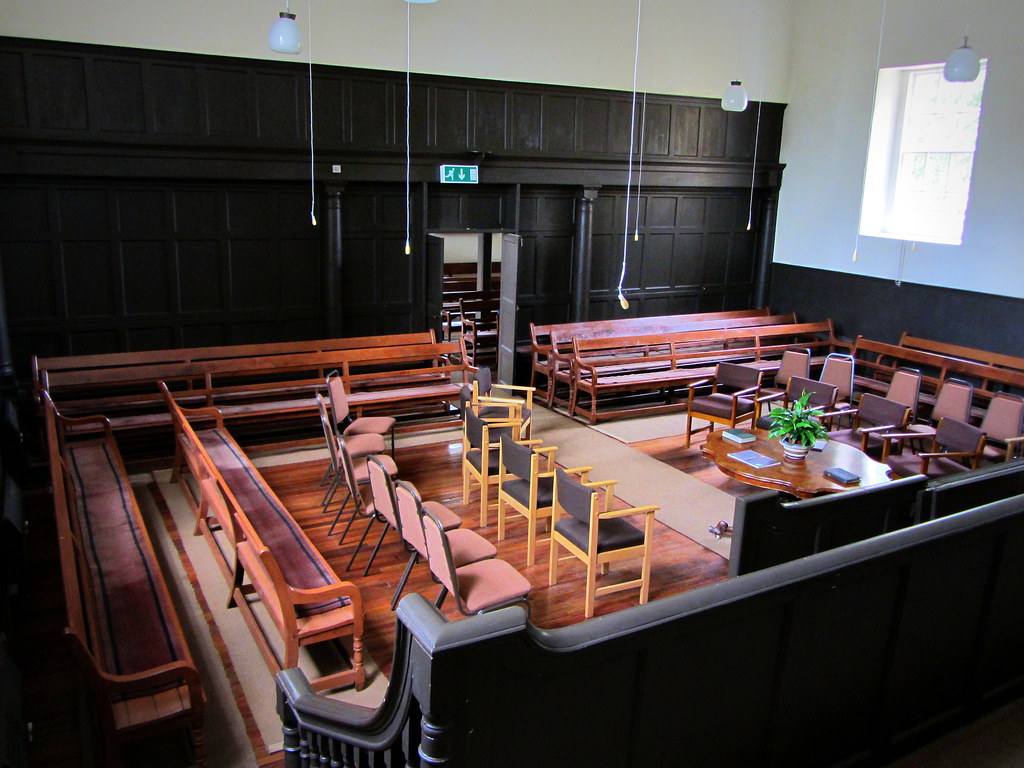This horizontal rectangular image depicts a spacious meeting room or academic setting characterized by an array of seating options and meticulous organization. The room features white or cream-colored walls and ceilings, complemented by a brown wooden floor. Along the back wall, which includes a mix of cabinets and a black door with an exit sign, there are wooden benches situated below hanging microphones. 

To the right, a large window allows natural light to flood the space, contrasting with lights and lamps hanging from the ceiling. In the center of the image, an oval or fish-shaped wooden coffee table holds a green plant and several books. Surrounding this table are curved rows of chairs—some with orange seats and backs, others being wooden chairs with cushioned seats and arms. 

Toward the left side of the room, there are additional benches and rows of chairs in various colors including brown, black, tan, yellow, and pink. Subtle details such as the intricate arrangement of seating, the daylight streaming through the window, and the overall blend of functional and aesthetic elements suggest an organized and inviting atmosphere, potentially one designed for collaborative or educational purposes.